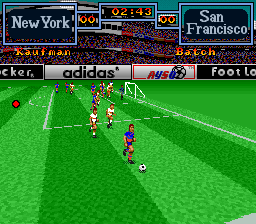This image is a screenshot from a retro soccer-themed video game. The visual perspective is from behind the goalpost, capturing players moving towards the camera slightly to the right. In the foreground, a goalpost is positioned centrally on the right side of the image. The game field extends into the background where numerous pixelated players can be seen dispersed across the pitch. The stadium surrounding the field is visible, complete with advertising banners lining the walls that separate the seating area from the playing field. The stadium's structure, though pixelated, is detailed enough to suggest a classic animated design characteristic of vintage gaming.